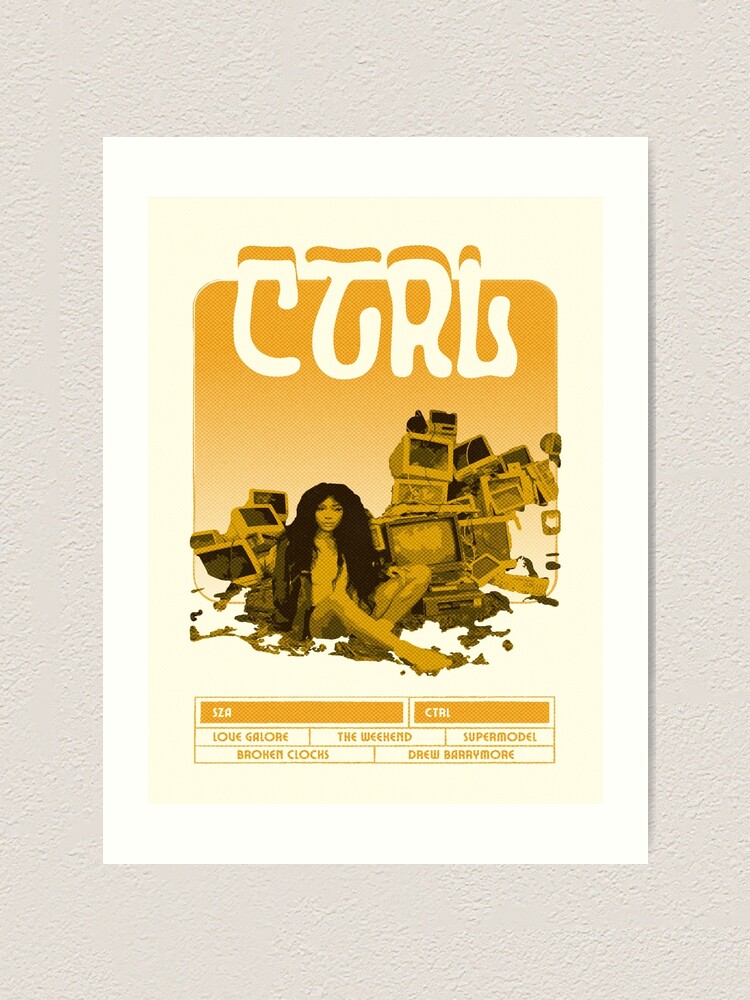The photograph depicts a poster displayed against a textured, off-white wall. The poster is printed on white paper with a peach-colored center. It features a prominent image of a woman, likely the singer SZA, with long black hair, sitting cross-legged on the ground in front of a pile of old computers and monitors. At the top of the poster, the word "CTRL" is written in bold white letters. Below the image, there are text boxes with orange bands labeled "SCA" and "CTRL." In a white text box beneath these, several song titles are listed in orange text: "Love Galore," "The Weeknd," "Supermodel," "Broken Clocks," and "Drew Barrymore." The design of the poster prominently features a palette of cream, orange, and black tones.